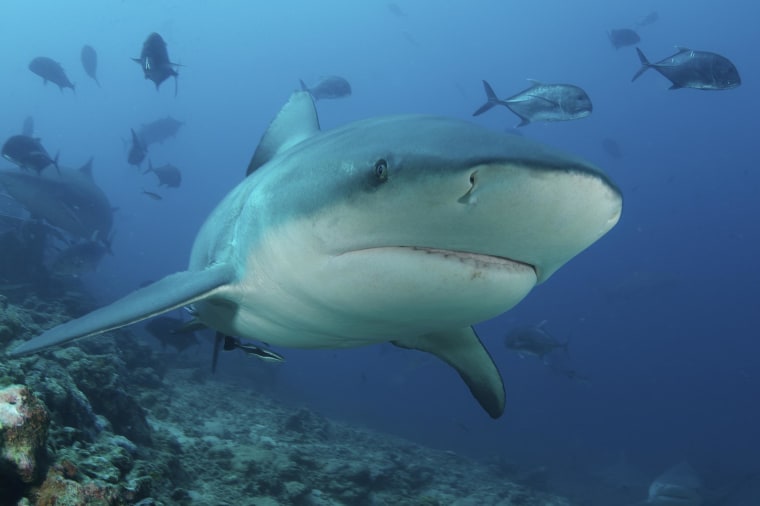This is a detailed, horizontal underwater photograph featuring a quintessentially recognizable shark, the stereotypical image one might imagine when thinking of a shark. The shark is swimming towards the camera, emerging from the left side and moving towards the right of the frame. Its mouth is closed, with the lower part of the mouth and nasal slits faintly visible beneath its body. The shark displays a classic color pattern: its underside is predominantly white or light gray, while the upper side features a darker grayish-blue hue, the division of which runs along the bottom side.

Prominent in the foreground, the shark’s right pectoral fin and dorsal fin are clearly visible, while its tail fin is obscured behind its body. Surrounding the shark are various smaller fishes; notably, two silvery blue fish are positioned just above its nose, swimming to the right, and several darker, less detailed fish reside in the background.

The photo's backdrop is a murky blue aquatic environment, presenting an array of marine life. Additionally, some dolphin fish, grouper fish, and other small fish are swimming around, creating a lively underwater scene. In the lower-left corner, the image reveals a reef with rocks and coral growth, extending from the upper part downward. In the far right-hand corner, a second, much smaller shark is visible, adding depth to the image.